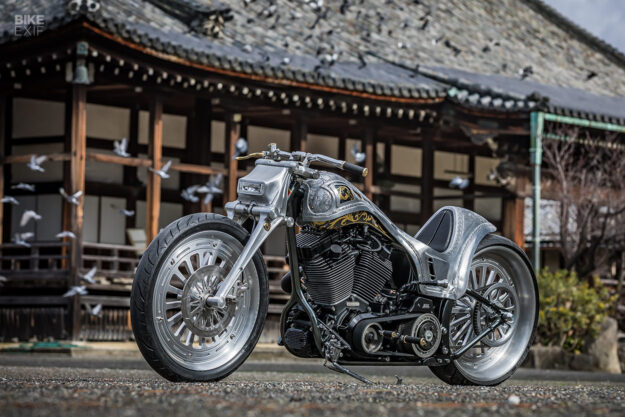The image depicts a highly customized, gothic-looking motorcycle with large wheels, primarily silver and charcoal gray, parked on a gravel road outside a traditional Asian building, likely inspired by Chinese or Japanese architecture. The building features wooden elements, including a porch and scaffolding, and characteristic upward-curving roofs. In the background, a flock of white birds is taking off, adding a dynamic element to the scene. The setting appears outdoors, and there is noticeable shrubbery around the area. The motorcycle stands out with its sleek design and short handlebars, contrasting with the ancient aesthetic of the building behind it. The overall impression is that of a meticulously crafted image, possibly photoshopped or AI-generated, blending modern mechanical artistry with historical architecture.